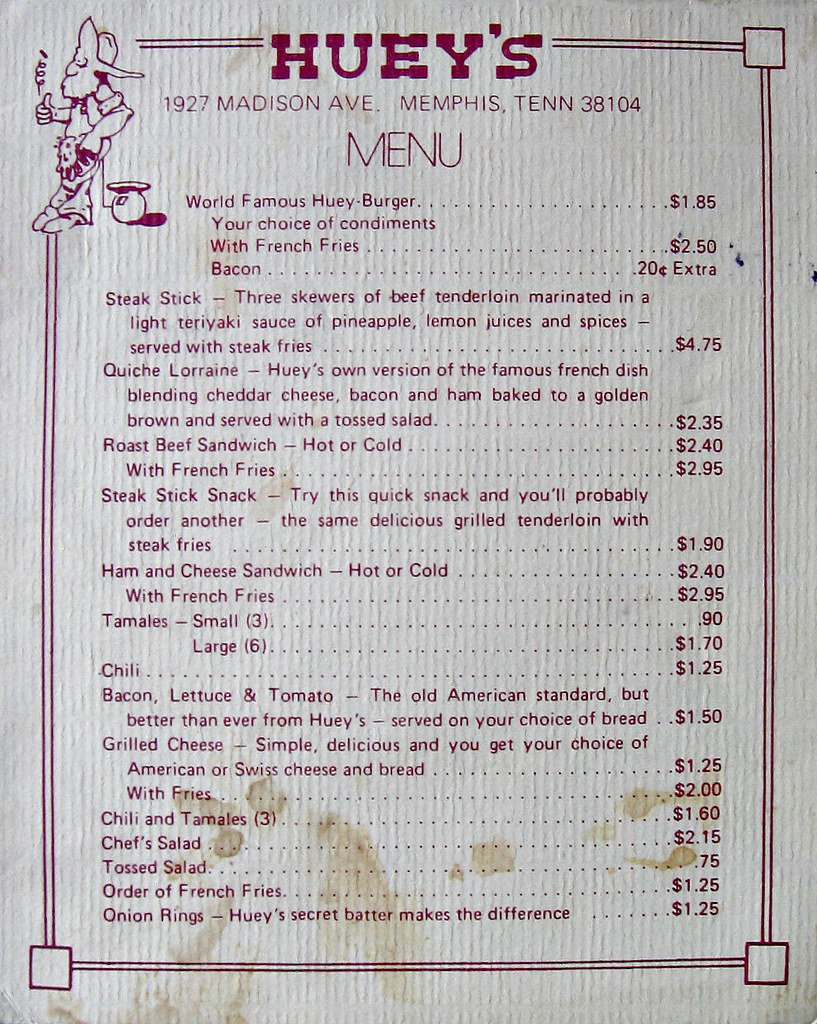The image is of a vintage restaurant menu set against a white background, with text written in a distinctive reddish-brown color. The menu is framed by an elegant border that encapsulates the offerings within. At the top, the menu reads "Huey's, 1927 Madison Avenue, Memphis, Tennessee, 38104," followed by the title "Menu." 

Adding a whimsical touch, there is an illustration to the left of this title: a man in a cowboy hat, casually leaning against the menu itself, flipping a coin. He exudes a relaxed demeanor, with one leg crossed over the other as he stands.

The menu presents an array of delectable items:
- "World Famous Huey Burger" for $1.85, with a choice of condiments. Adding French fries raises the price to $2.50, while bacon adds an extra $0.20.
- "Steak Stick," featuring three skewers of beef tenderloin marinated in a light teriyaki sauce composed of pineapple, lemon juices, and spices, served with steak fries for $4.75.
- "Quiche Laurent," Huey's unique take on the French classic, combining cheddar cheese, bacon, and ham, baked to golden perfection and accompanied by a tossed salad for $2.35.
- "Roast Beef Sandwich," available hot or cold for $2.40, or with French fries for $2.95.
- "Steak Stick Snack," a quick version of the grilled tenderloin with steak fries for $1.90.
- "Ham and Cheese Sandwich," hot or cold, priced at $2.40, with an option to add fries for $2.95.
- Tamales are offered in different portions: three small for $0.90 or six large for $1.70.
- "Chili" is available for $1.25.
- "Bacon, Lettuce, and Tomato" sandwich, a refined take on the classic, served on your choice of bread for $1.50.
- "Grilled Cheese," available with American or Swiss cheese and your choice of bread, for $1.25, or with fries for $2.
- "Chili and Tamales," featuring three tamales for $1.60.
- "Chef’s Salad" for $2.15.
- "Tossed Salad" for $0.75.
- "Order of French Fries" for $1.25.
- "Onion Rings," enhanced by Huey's secret batter, for $1.25.

The menu shows signs of wear, with smudges of sauce at the bottom and vertical ridge lines running from top to bottom, adding a touch of nostalgia to this charming document.